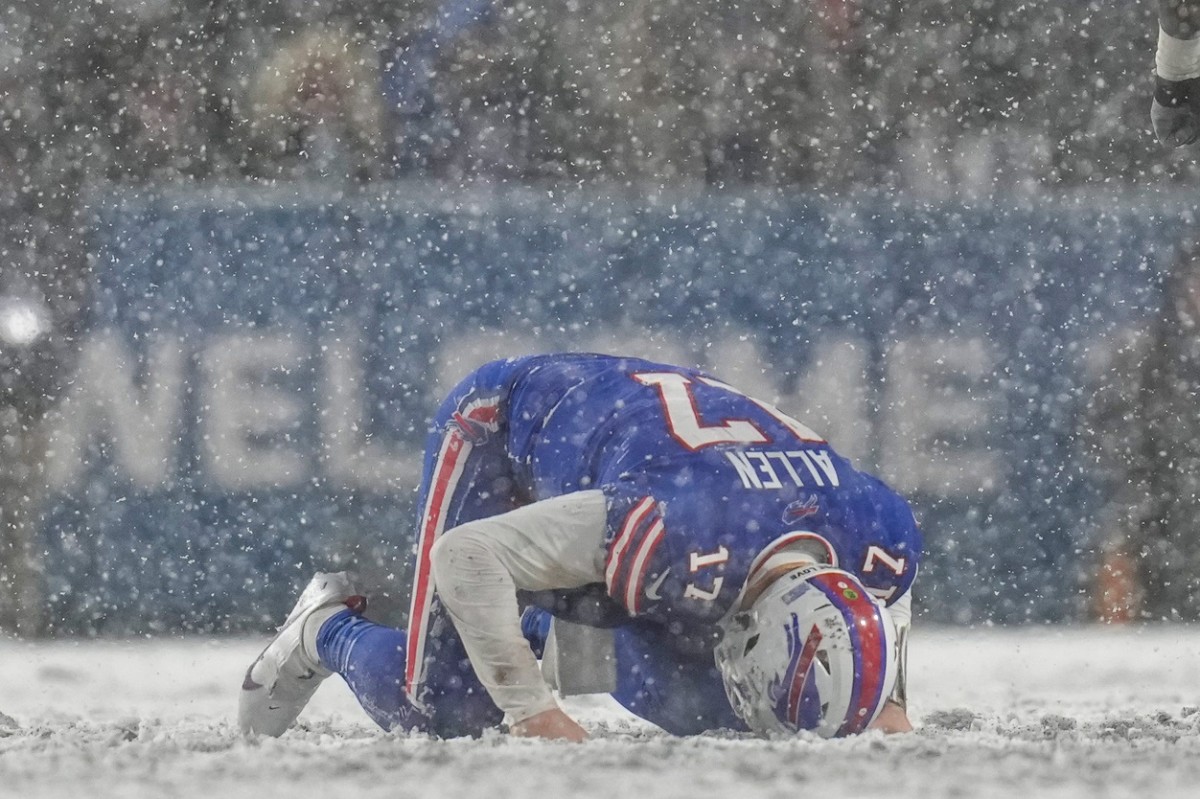In this photograph, taken outdoors during a snowfall, a football player is featured on a snowy field. The dense snowfall gives the entire image a foggy appearance. The ground is covered in a thick layer of white snow, and the falling snowflakes are prominently visible. 

The player is on his knees with his head bent down, touching the ground. He is wearing a blue football uniform with red and white stripes running down the legs of his pants and across his shoulders. His jersey has the name "ALLEN" in white letters and the number "17" in white, outlined in red. He also sports a white helmet adorned with a blue design and a red stripe down the middle. Underneath his jersey, he wears a white long-sleeve shirt, and his white cleats feature a black Nike logo.

In the background, partially obscured by the falling snow, there is a large blue banner with the word "WELCOME" written in white letters. This banner stretches across the middle of the image, adding depth to the scene.